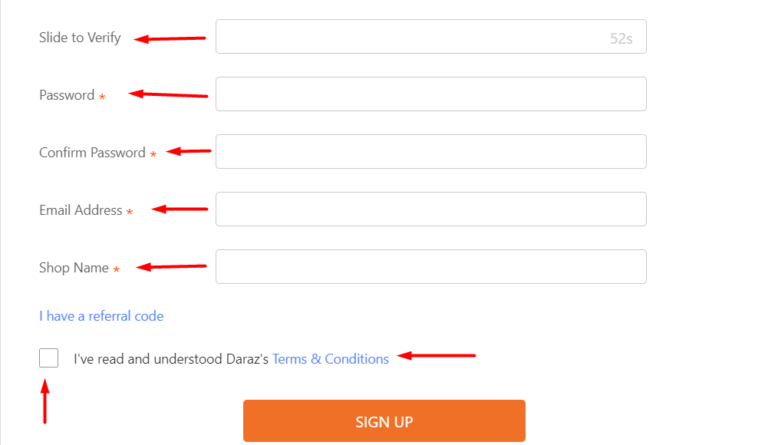Here is a refined and detailed caption:

---

This image is a screenshot of a user registration form featuring several input fields and annotations indicating potential edits. The form's background is white, with light gray outlines marking the input boxes for a minimalistic design. Red arrows point from each input box to their corresponding titles, suggesting that these elements may need to be moved closer together. 

1. The first section, labeled "Slide to verify," has an associated text box containing the placeholder "52S."
2. The next field is "Password," marked with a red asterisk to denote it as a required field. An input box is placed next to it, with an arrow pointing between the two elements.
3. "Confirm Password" follows, also marked with a red asterisk, indicating it is mandatory. Similarly, a red arrow connects the title to its respective input box.
4. The "Email Address" field is next, complete with a red asterisk and an accompanying arrow pointing to the input box.
5. Lastly, "Shop Name" is listed with a red asterisk, followed by an arrow directed at its input box.

Below these input fields, in blue text, is the optional "I have a referral code" checkbox. Beneath this is another checkbox labeled "I've read and understood the RAS's T's and C's," with "terms and conditions" highlighted in blue text.

This annotation suggests a structural adjustment to make the form more user-friendly by aligning the input boxes closer to their labels.

---